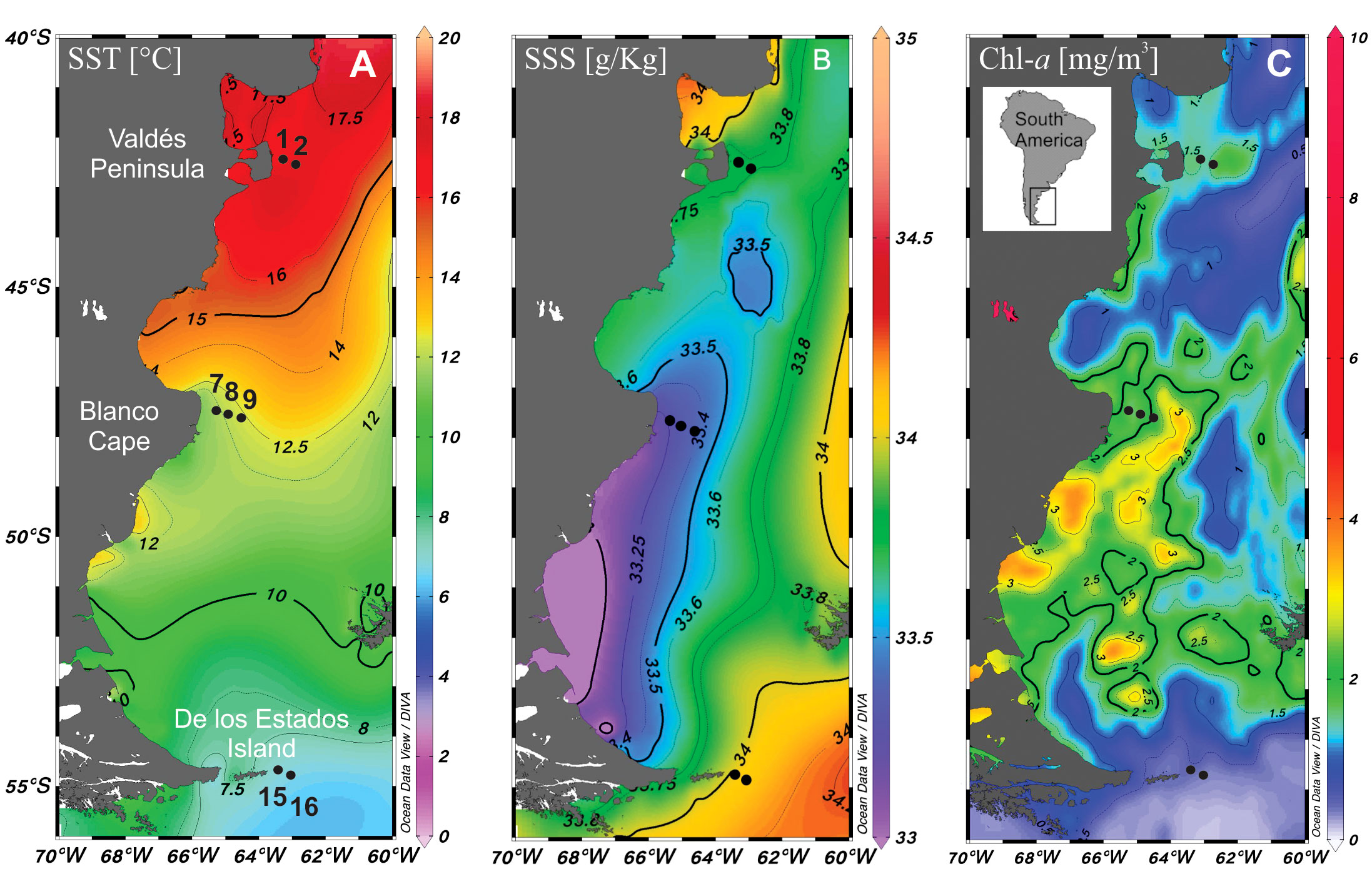The image comprises three vertically aligned sections, each depicting the same landmass—a portion of South America's lower region, particularly near the Valdez Peninsula off the coast of Argentina. Each section is a detailed map overlaid with color gradients representing different measurements. The maps are labeled A, B, and C.

Map A, labeled "SST (°C)," shows sea surface temperature in degrees Celsius. The temperature ranges from 0°C to 20°C, represented by colors from purple (coldest) to red (hottest).

Map B, labeled "SSS (g/kg)," displays sea surface salinity in grams per kilogram. It uses a different color gradient but follows a similar visual scheme.

Map C, labeled "CHL-a (mg/m³)," illustrates chlorophyll-a concentration in milligrams per cubic meter, indicating the presence of phytoplankton.

Each map includes labels for key geographic locations such as Valdez Peninsula, Blanco Cape, and De Los Estados Island. The left side of the maps features latitude lines ranging from 40°S to 55°S, and the bottom of the maps displays longitude lines from 70°W to 60°W. The right side of each map includes a color key corresponding to the respective measurement's range. A smaller inset in gray also highlights South America, contextualizing the specific region being analyzed.